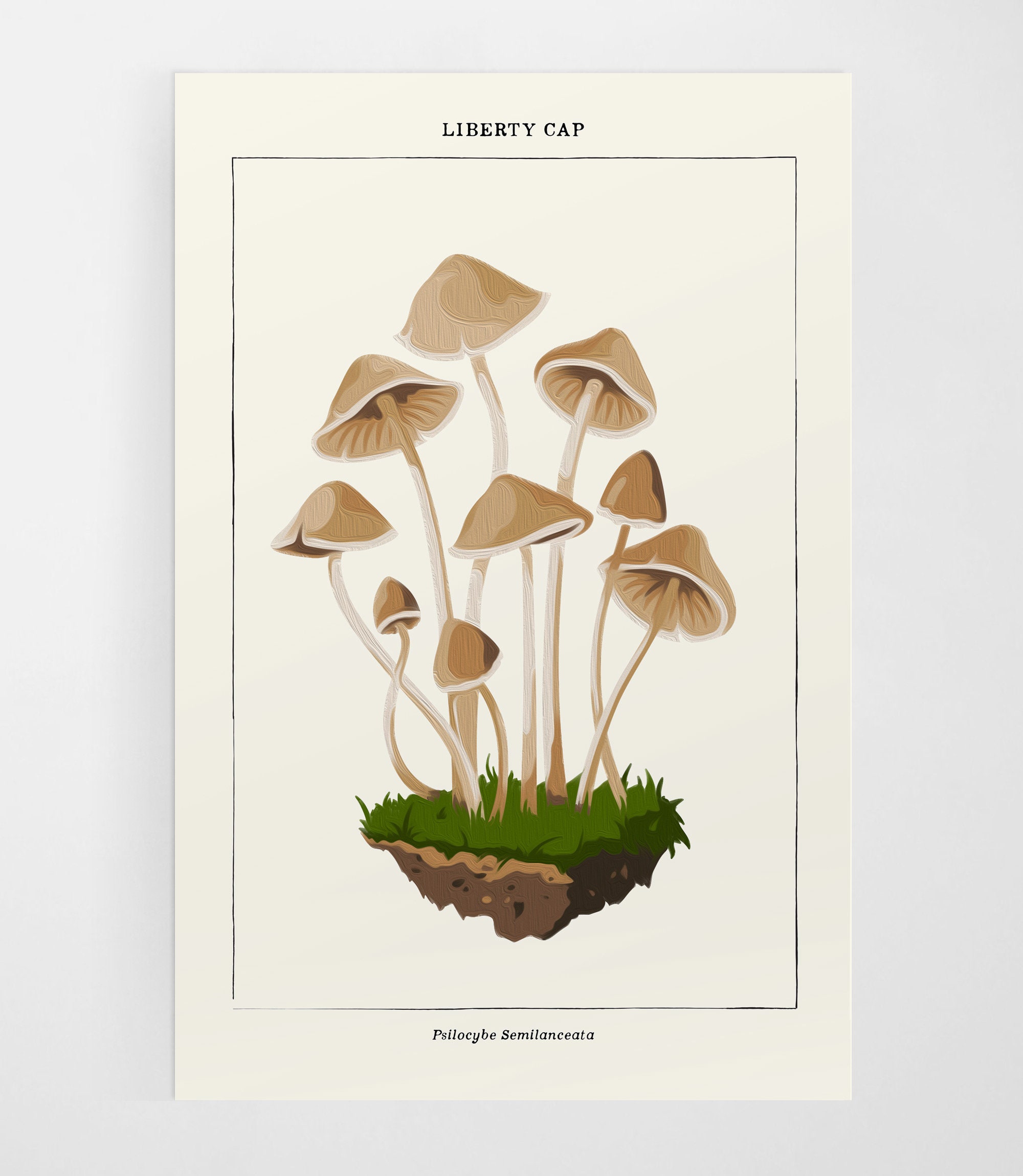The image is a detailed vertical illustration of the Liberty Cap Mushroom against an off-white, tan cream background, framed by a light black rectangular outline. At the top center, in dark, capitalized lettering, it reads "Liberty Cap," and at the bottom, it is labeled with the Latin species name "Psilocybe similacata." The illustration prominently features a cluster of ten Liberty Cap Mushrooms, each with distinctive, tall, thin white stalks and light brown to tan bell-shaped caps, some of which are positioned to display the intricate gill lines on their undersides. The mushrooms vary in height and angle, with three smaller, more conical ones amidst the group. They emerge from a patch of green, spiky grass rooted in a chunk of brown, textured soil, implying a natural setting where these mushrooms grow. The meticulous details of the earthy base, along with the varied angles and heights of the mushrooms, vividly depict the characteristic appearance of the Liberty Cap Mushroom.